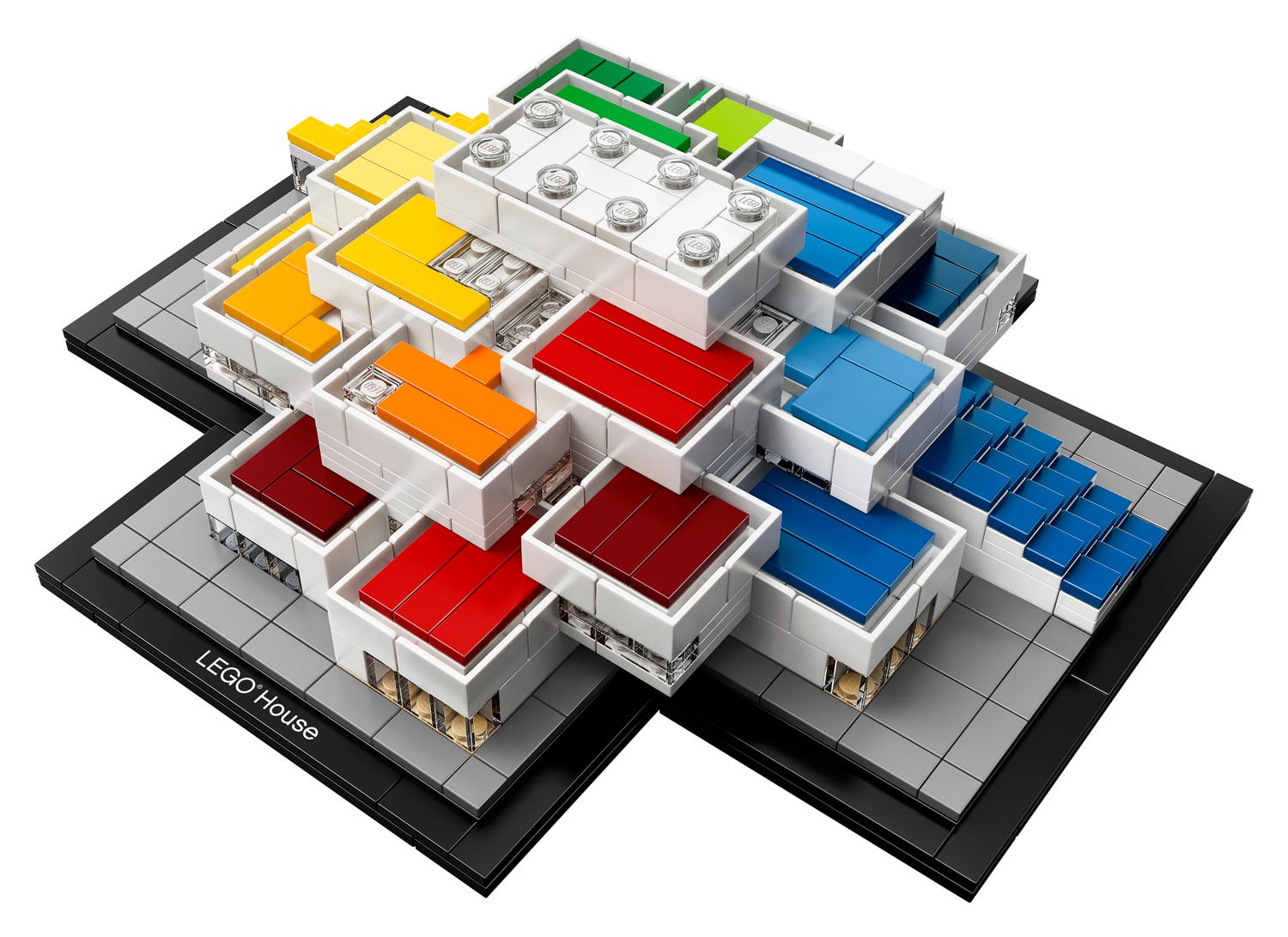The image showcases a detailed Lego house model built with an assortment of colorful Lego bricks. The structure features a vibrant array of colors including dark blue, light blue, red, orange, yellow, green, and brown, creating a striking visual appeal. The house stands on a gray platform which is mounted on a black base. The black base extends in a T-shape, with the words "Lego House" prominently displayed in white lettering on one side. The roof sections of the house are particularly colorful, utilizing a mix of dark red, orange, yellow, green, and varying shades of blue. At the very top, a white two-by-four Lego brick is visible, adding a unique detail to the model. The entire composition is set against a white background, presented at an axonometric angle which gives a three-dimensional perspective to the house. This Lego model appears to be professionally constructed and may represent a prototype for an actual building, with most traditional Lego connectors hidden, allowing for a sleek and polished appearance.